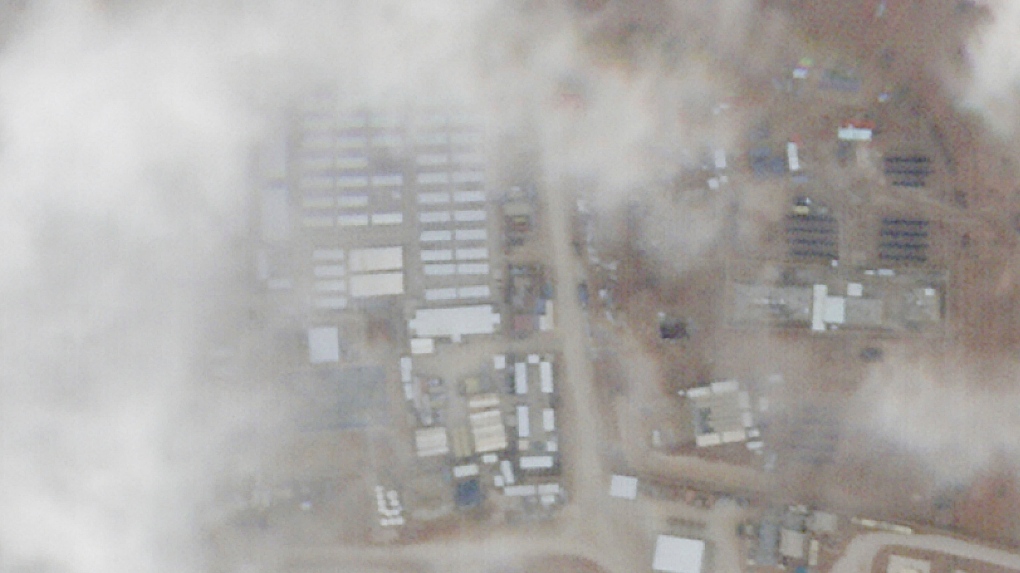This horizontally rectangular, color aerial photograph taken during the daytime provides a detailed overhead view from an airplane perspective, looking down through the clouds onto an industrial complex or city. The scene is dominated by a blanket of clouds, especially thick on the entire left side of the image, thinning towards the center and right. Nestled among these clouds, the ground below reveals several buildings and a network of roads threading through them. These edifices, primarily white and black in color, appear as a mix of rectangular shapes—potentially buildings or shipping containers—with those on the left being more white and orderly, while those on the top and middle right are darker. Additionally, faint dirt roads trace a path from the very top center downward, interspersed with other pathways. The overall setting is starkly monochromatic, with the white and gray of the clouds juxtaposed against the earthly browns and grays of the roads and buildings. High above, any specific details like people or vehicles remain indiscernible, though small, stretched-out white shapes near the top right could possibly be semi-trucks. This overhead photograph captures a slice of industrial or urban landscape through a veil of clouds, offering a unique top-down perspective.